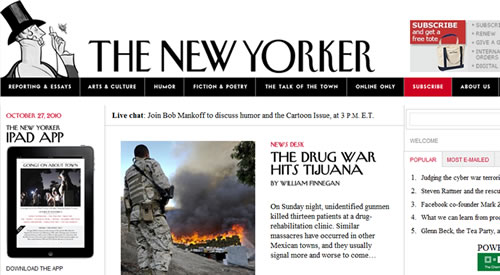This is a detailed screenshot of the New Yorker website, captured in landscape mode on a desktop. The header features the iconic New Yorker logo, depicting a man in a high-brimmed shirt and top hat, holding a monocle, rendered in black and white, located at the top left corner. Centrally located at the top is the bold text, "The New Yorker." On the top right corner, a promotional banner reads, "Subscribe and get a free tote," accompanied by an image of a tote bag against a dual gray and red background, with a noticeable red subscribe button.

Just below the header, a navigation bar extends across the page, listing various sections: "Reporting," "Arts and Culture," "Humor," "Fiction and Poetry," "The Talk of the Town," and "Online Only." A red subscribe button and an "About Us" link are also present at the end of the navigation options.

On the lower left side of the page, there's information about the New Yorker iPad app, dated October 27th, 2020. This section includes an image of an iPad displaying text and a button that prompts visitors to download the app.

Centrally situated on the page is a live chat feature. Below this, there is a section labeled "News Desk," highlighting a story titled "The Drug War Hits Tijuana," accompanied by a photograph of a soldier and a burning drug field, followed by descriptive text.

On the right side, a welcome message is displayed above a white search bar. Beneath the search bar is a list of popular stories, ranked from one to five. The entire webpage is set against a clean, white background, presenting the information in a clear and organized manner.